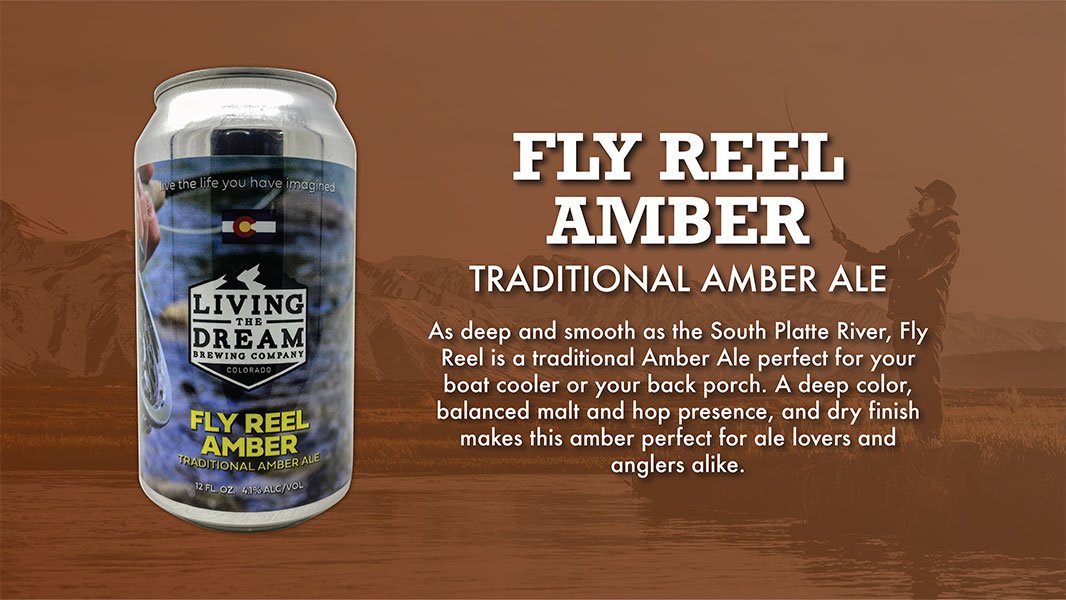This image is an advertisement for Fly Real Amber, a traditional amber ale by Living the Dream Brewing Company. In the foreground, a silver 12-fluid ounce can of the ale is prominently featured on the left side. The can's label is designed with blue and brown colors, and it reads: "Living the Dream Brewing Company Colorado. Fly Real Amber Traditional Amber Ale." Accompanying text further describes the ale: "As deep and smooth as the South Platte River, Fly Real is a traditional amber ale perfect for your boat cooler or your back porch. Its deep color, balanced malt and hop presence, and dry finish make it ideal for ale lovers and anglers alike." In the background, a blurred fishing scene features a fly fisherman in a jacket and hat, set against a backdrop of mountainous terrain, encapsulating the rugged, outdoor vibe of the brand. The overall color palette of the image is a mix of vibrant hues contrasting with the subtle, natural tones of the background.